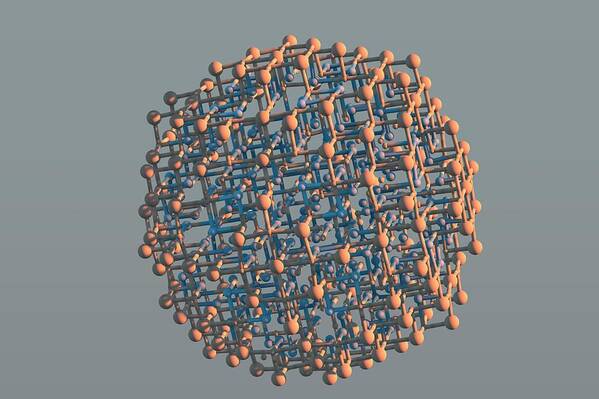The image is a visually striking piece of art set against a medium gray, horizontally oriented rectangular backdrop. At the center of the image is a large, round structure reminiscent of a geodesic dome, constructed from interconnected elements that resemble plane jacks. The spherical form appears to be crafted from numerous knobs and lines, which intertwine both inside and outside the structure. The outer part of the sphere is predominantly orange, while the inner portion showcases a vivid mix of blue, black, and purple hues. The various connecting pieces and smaller dots within the structure add to its intricate and complex appearance, suggesting it could either represent a scientific model or purely artistic creation.